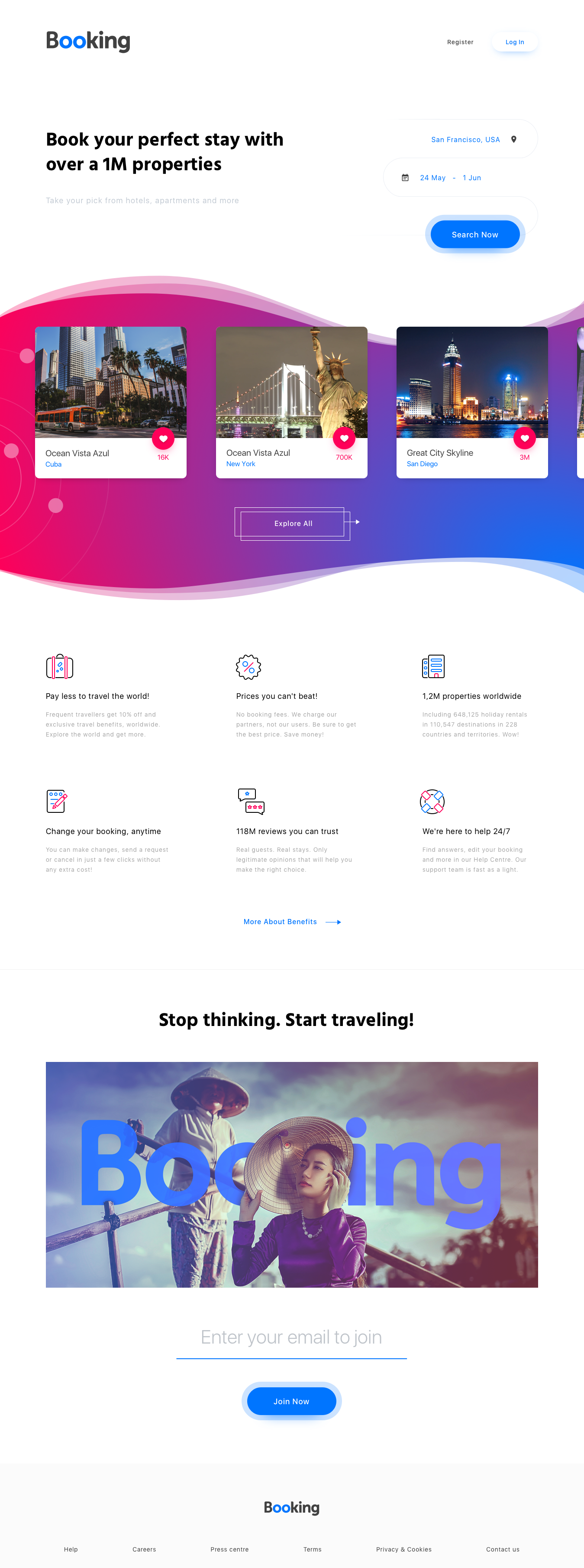Here is the refined and detailed caption:

---

The screenshot depicts a Booking.com landing page tailored for potential renters seeking accommodations. In the top left corner, the familiar Booking.com logo is prominently displayed, with "Register" and "Login" options visible to the right. The main call-to-action text reads: "Book your perfect stay with over 1 million properties." On the left side, a search prompt specifies "San Francisco, USA" and the dates "from the 24th of May to the 1st of June," encouraging users to choose among various lodging types, including hotels and apartments.

The center section of the page features explore options such as "Ocean Vista Azul in Cuba," "Ocean Vista Azul in New York," and "Great City Skyline in San Diego." Below this is an array of icons and promotional statements: an illustration of a suitcase beside "Pay less to travel the world," a squiggly circle with a percentage sign and "Prices you can't beat," two drawings of apartment buildings with "1.2 million properties worldwide," a paper with a pencil and "Change your booking any time," and two speech bubbles near "108 million reviews you can trust." Additionally, a life book icon is accompanied by "We’re here to help 24-7."

Toward the bottom of the page is an invitation for users to join by entering their email, paired with the encouraging slogan, "Stop thinking, start traveling."